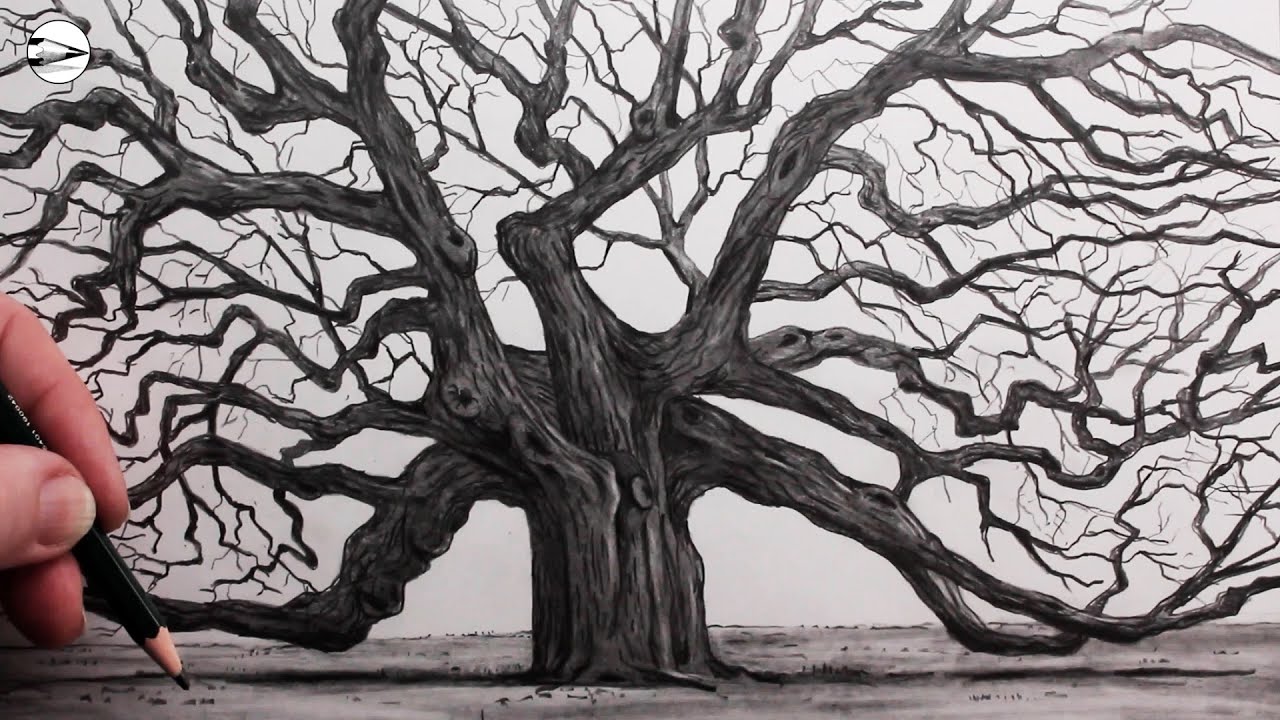The image captures the detailed black and white drawing of a large, old, gnarled tree with no leaves, its many crooked branches sprawling in all directions, some even touching the ground. The tree, reminiscent of a Halloween or horror movie scene, has a thick trunk and exudes an eerie, ancient presence as if it could be a hundred years old. In the backdrop, there is a faint outline of the moon or sun adding to the spooky atmosphere. In the bottom left corner of the photo, a left hand holding a pencil is visible, suggesting the artist is either finishing up or has just completed this incredibly realistic and artistically detailed sketch.